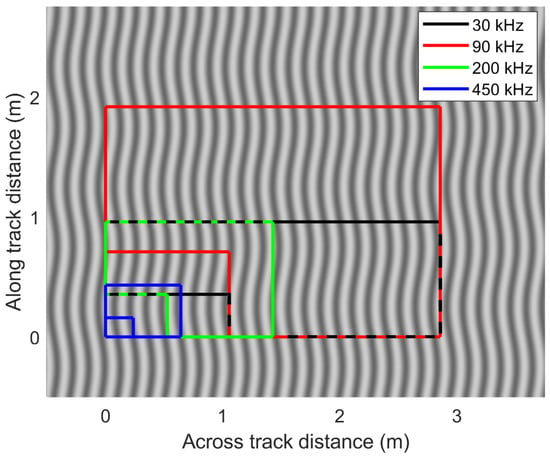The image represents a detailed sound wave analysis graph. The graph has a Y-axis labeled "along track distance (M)" and an X-axis labeled "cross-track distance (M)". The Y-axis is marked from 0 to 2, while the X-axis ranges from 0 to 3. The background features wavy black lines on a gray field, resembling an optical illusion.

Within the graph are multiple colored rectangular boxes, each corresponding to different frequency measurements as indicated by a legend. The legend specifies:

- Black for 30 kHz
- Red for 90 kHz
- Green for 200 kHz
- Blue for 450 kHz

The boxes' outlines are defined by these colors, with some boxes nested within others, creating a layered effect. The smallest box, outlined in dark blue (450 kHz), is positioned near the coordinates (0,0). The black box (30 kHz) outlines the entire nested structure. The red boxes (90 kHz) are larger and span multiple areas, while the green boxes (200 kHz) encapsulate the red boxes. The positional and size-based relationships among the boxes provide a visual representation of the sound wave frequencies across different distances on the grid.